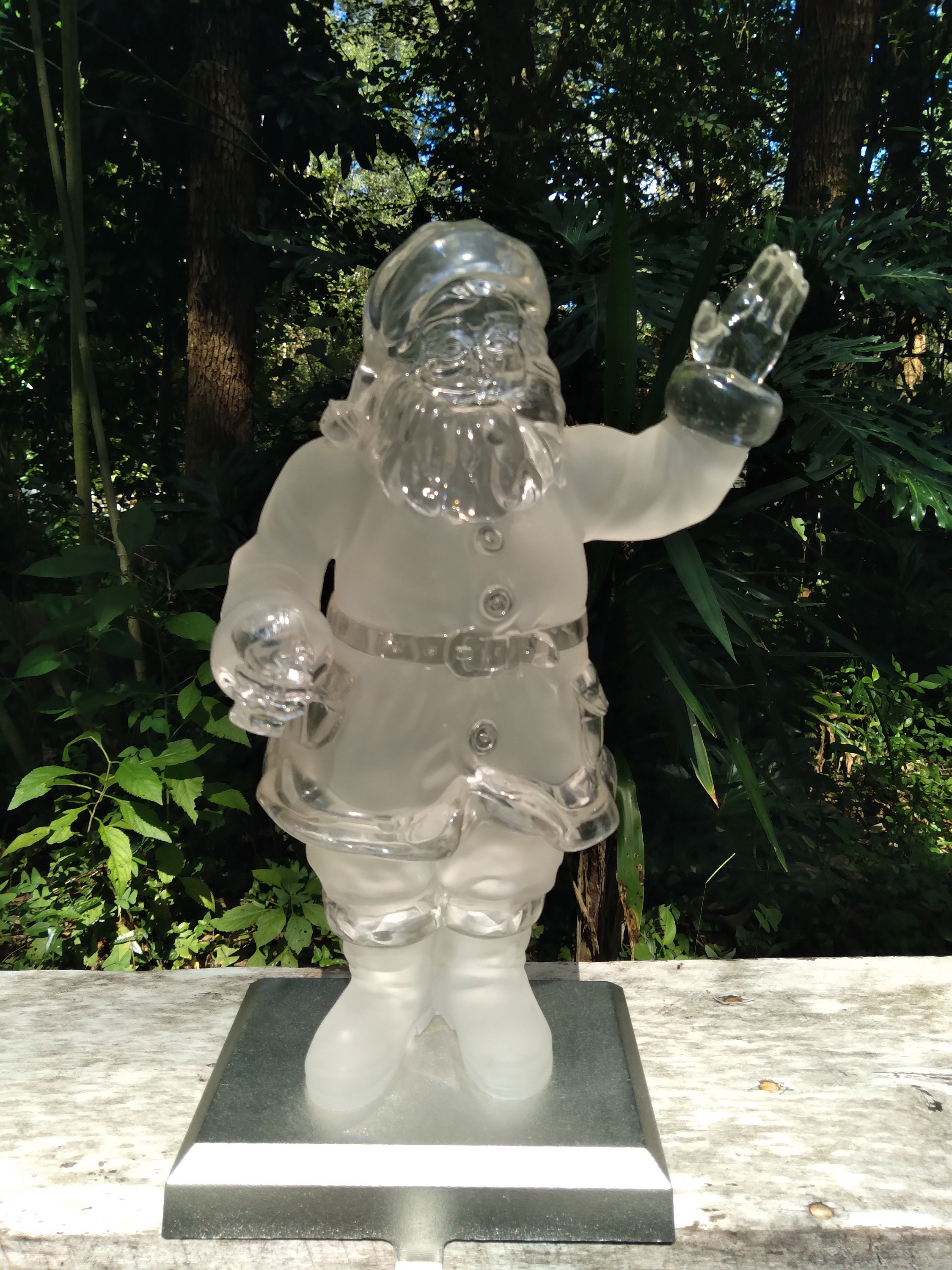The image captures a detailed view of an outdoor scene during the daytime, with a lush, green forest serving as the backdrop. Trees with brown trunks and dense foliage, along with various bushes and plants with large green leaves, create a rich tapestry of greenery behind the focal subject. In the foreground rests a small wall or bench made of a white and gray stone, upon which sits a reflective silver pedestal. Atop this pedestal stands a meticulously crafted statue of Santa Claus, seemingly made from either translucent crystal or glass, with parts of it appearing frosted to add texture. Santa Claus, depicted in his traditional outfit, complete with a heavy coat, a belt, long pants, and boots, has his left hand raised in a waving gesture. His beard, almost fully translucent, catches the light, and his cap, adorned with a bell at the end, illustrates his classic look. The craftsmanship of the statue, combined with its reflective qualities, contrasts beautifully with the natural elements surrounding it.